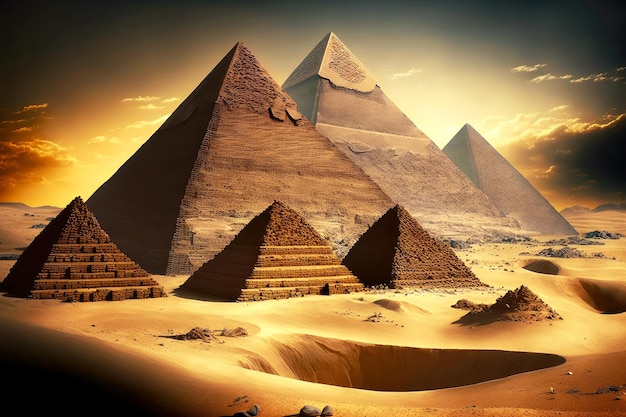This digital image captures a striking view of the pyramids in Egypt, likely taken during sunrise or sunset, as the sky transitions from dark at the top to a radiant ring of orange and yellow near the horizon. In the foreground, three aged and crumbling small pyramids sit on a sandy expanse, their tiered structures clearly visible. To the right, a conspicuous giant rectangular sand pit and an adjacent pile of dirt command attention. Behind these, three significantly larger pyramids rise prominently. The leftmost large pyramid has stones visibly falling off, while the pyramid in the middle boasts a smooth stone cap adorned with a symbol. The entire scene is suffused with a glowing yellow light that highlights the sand and the pyramids' brownish tones, intensifying the stark and almost surreal atmosphere. The background reveals the sun partially obscured behind one of the pyramids, casting a glow that illuminates the entire tableau.